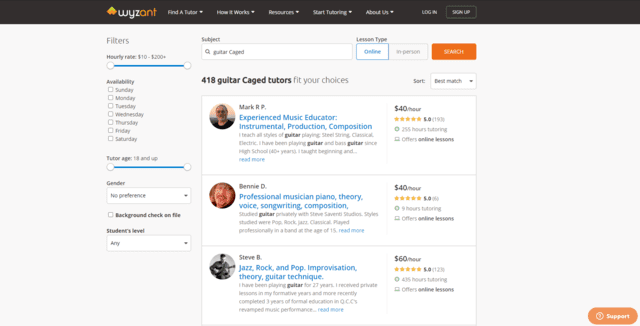The image features a light blue background. At the top, there's a black header containing the Wyzant logo. The "W-Y-Z" letters are in white, while the "A-N-T" letters are in orange. Next to the logo is a small orange insignia. The navigation menu includes options like "Find a Tutor," "How It Works," an indiscernible word, "Start Training," and "About Us," all with drop-down functionalities. On the right side of the header are the "Log In" and "Sign Up" buttons.

Below the header, there is a light blue section with various filters. At the top of this section, there is a label titled "Filters." The first filter is an hourly rate slider ranging from $10, marked by a small circle with a blue line and another circle. Following that, there's an availability filter, listing the days of the week each with a small checkbox. Below is an age filter labeled "Tutor Age 18 and Up," featuring two circles connected by a blue line.

Further options include a gender filter with a drop-down menu, a "Background Check on File" option with a checkbox, and a "Students Level" filter with another drop-down menu. On the right side, there's a "Subject" filter with a search or drop-down menu, followed by a "Lesson Type" section. This section includes two options: a blue-bordered white box labeled "Online" in blue text, and another box for "In-Person."

An orange search button at the bottom states, "418 guitar cage tutors fit your choices." This is followed by three tutor profiles, the first two charging $40 per hour and the third charging $60 per hour.